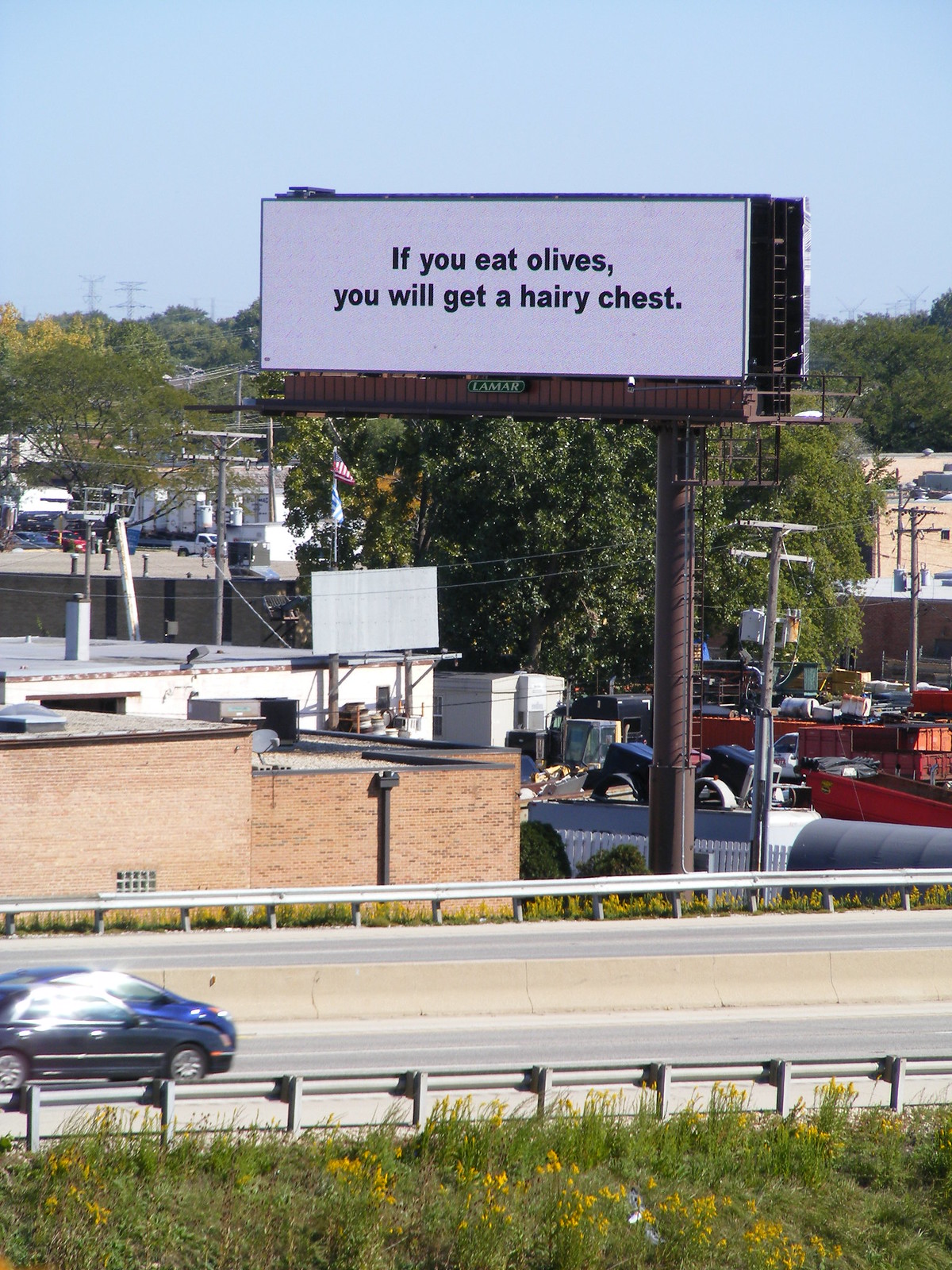This captivating photograph showcases a quintessential highway scene bordered by an array of elements that adds depth and detail to the composition. In the foreground, a lush strip of green grass sprinkled with bright yellow flowers leads the eye to a sturdy silver metal barricade. Beyond this barricade, the gray paved road stretches onwards, hosting a blue and a black car in the bottom left corner.

A concrete divider separates these two lanes from the opposite side, adding a structured feel to the roadway. On either side of the road, there is a mix of structures; to the front left, tan brick buildings stand prominently, complemented by a distant white building with a gray roof.

In the distance, more vehicles and verdant green trees scatter across the scene, hinting at the perpetual motion of urban life. A brown metal cylinder supports a billboard, its intricate design featuring a walkway labeled "Lamar" in green lettering. Contrasting against the backdrop, the white billboard boldly declares in black print, "If you eat olives, you will get a hairy chest," adding a touch of humor to the lively tableau.